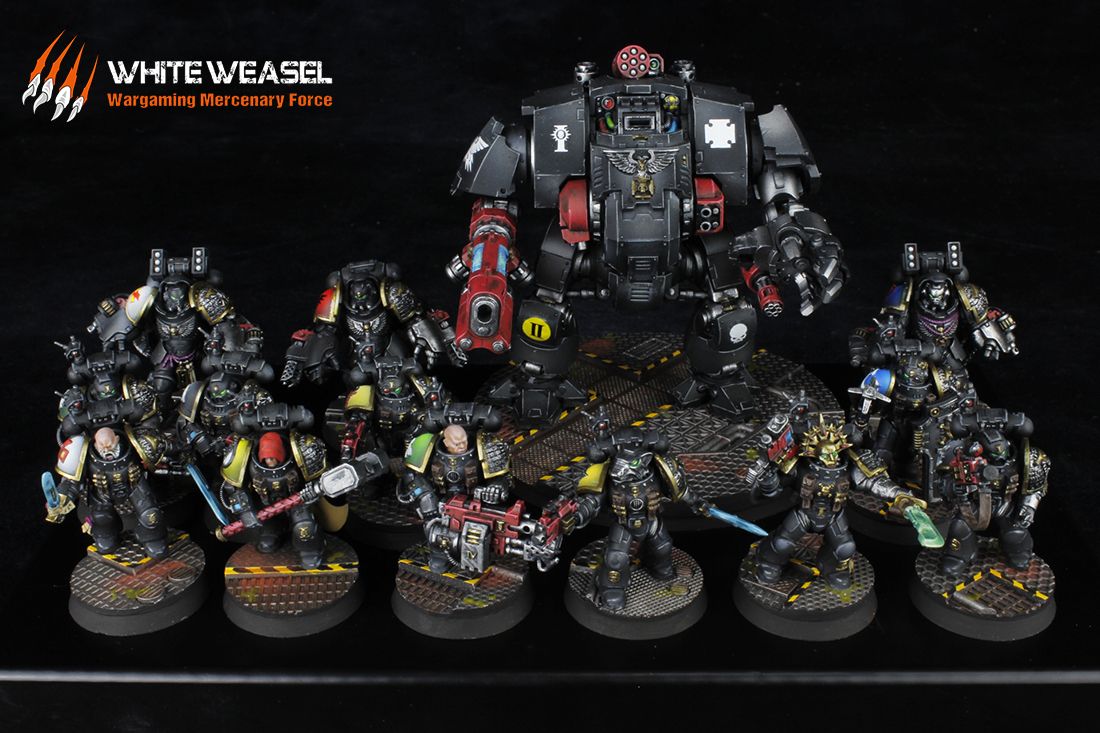In this landscape-mode photograph featuring a black background and a black table, a collection of intricately designed fantasy sci-fi figurines is displayed. Each figurine stands upright on a puck-like disc, serving as a base. The figurines vary in their armor, shapes, and appearances, representing an assortment of creatures or robot suits, with some suits closed, obscuring the wearer’s identity. Dominating the middle background is a notably larger figurine, shaped like a giant robot suit. This imposing figure wields a large gun as its right arm, which is colored red, and has a significant hand on the other. Positioned in the top left corner of the image are the words "White Weasel Wargaming Mercenary Force" in red letters, accompanied by an icon of four red claws with white talons. This detailed setting suggests an advertisement for a collection of alien-looking, robot fighters, highlighting the taller robot's distinct size and armament amidst its diverse companions.